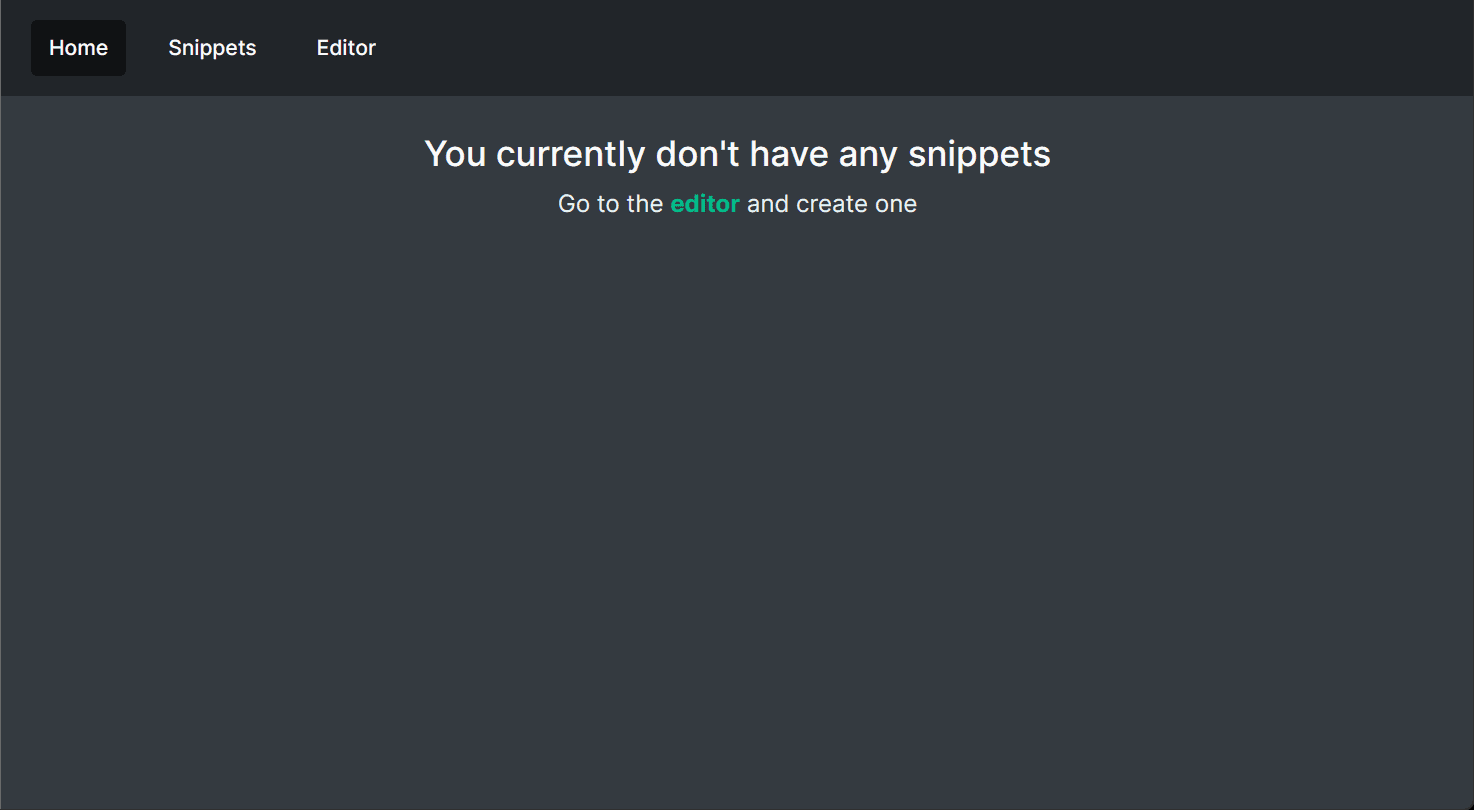This is a screenshot of a software application interface in landscape orientation. The top section features a black bar with three tabs, each labeled in white text— "Home," "Snippets," and "Editor." The "Home" tab, located in the top left corner, is highlighted in a darker black shade, indicating it is currently selected.

Below this black bar is the main screen, which is a lighter shade of dark gray than the bar itself. The main screen features two lines of text. The first line is in white, stating, "You currently don't have any snippets." The second line of text reads, "Go to the Editor and create one," with the word "Editor" emphasized in green. The overall interface utilizes a minimalist design with white text on various shades of dark gray and black backgrounds, emphasizing function over form.